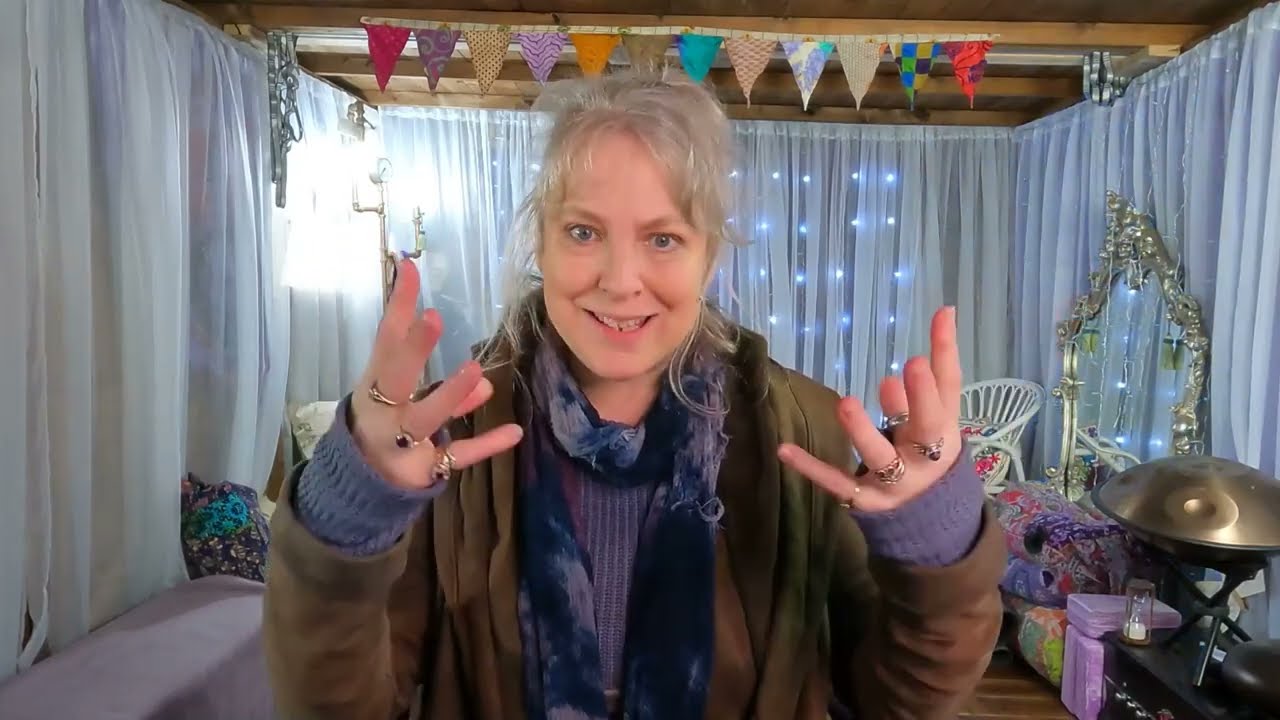The image depicts a Caucasian woman with light blonde hair, blue eyes, and a pale complexion. She is slightly off-center, glancing directly at the camera with her mouth open, suggesting she is in mid-speech, possibly of a spiritual or mystical nature. She wears layered clothing, comprising a blue and white scarf, a purple sweater, and a greenish-brown jacket, accessorized with rings on every finger.

The setting is a room infused with a spiritual ambiance, rich in colors and intricate decor. Behind her, white drapery extends around the space, complemented by exposed light wooden beams overhead. A banner featuring vibrant triangles in shades of red, blue, orange, purple, tan, and green hangs across the top of the image. To her right, there is a gold-framed mirror, a gold round object, a samovar-type structure, and a white chair with colorful draping. On her left, a lavender bench adorned with purple pillows is visible.

The room's furniture and decor exude an eclectic mix of purples, blues, oranges, and golds, creating a lively and mystical background. Small white lights dot the backdrop, enhancing the enigmatic atmosphere of the space. The overall composition and the woman's pose insinuate she may be engaged in a spiritual address or fortune-telling session, amplifying the image’s mystical and introspective aura.